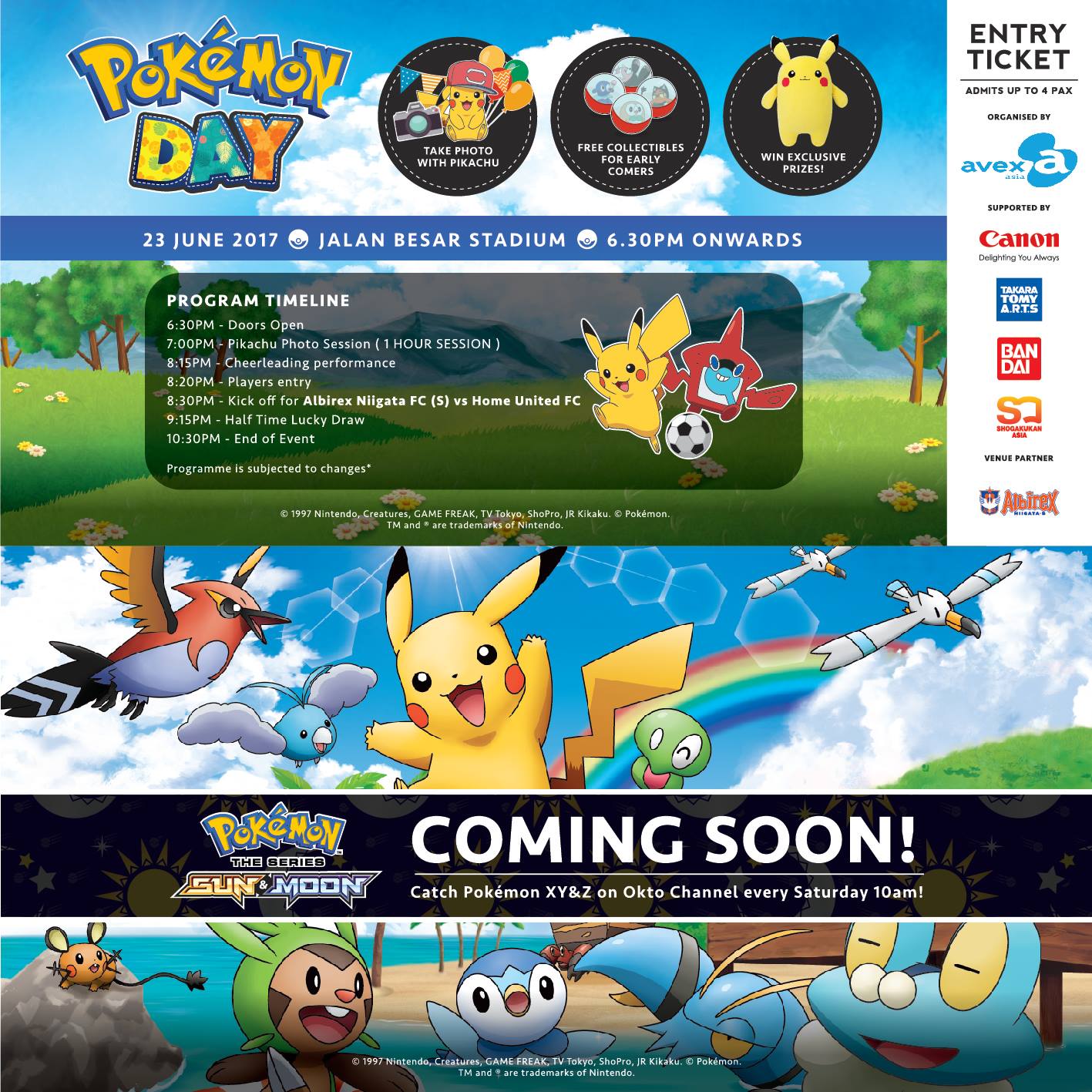In this vibrant and engaging image, we are presented with a dynamic Pokemon-themed website. At the top left corner, the words "Pokemon Day" are displayed prominently in bold letters, with each letter of "Day" in a different color, adorned with small explosions and decorations enhancing the festive feel. "Pokemon" is spelled in yellow. 

To the right of this heading, the website invites visitors to "Take a photo with Pikachu," featuring an image of the beloved character. Continuing to the right, there's a mention of some sort of free getaways, followed by information enclosed in a circle about exclusive prizes, specifying the event date as "23rd of June 2017" at the Jolene Bazaar Stadium, starting from 6:30 p.m. onwards.

Below this, the website features a program timeline including various Pokemon characters, and an itinerary detailing the events from 6:10 p.m. to 10:30 p.m. In a large rectangular section below this itinerary, the site showcases six Pokemon characters, including a prominent image of Pikachu in the center, overlaid with white text that announces, "Coming Soon: Catch Pokemon X, Y, & Z on Octo Channel every Saturday at 10 a.m."

To the left of this section, there's a mention of "Pokemon Sun and Moon." Beneath this, in another large rectangle, five additional Pokemon characters are displayed, adding to the excitement and visual appeal of the website.